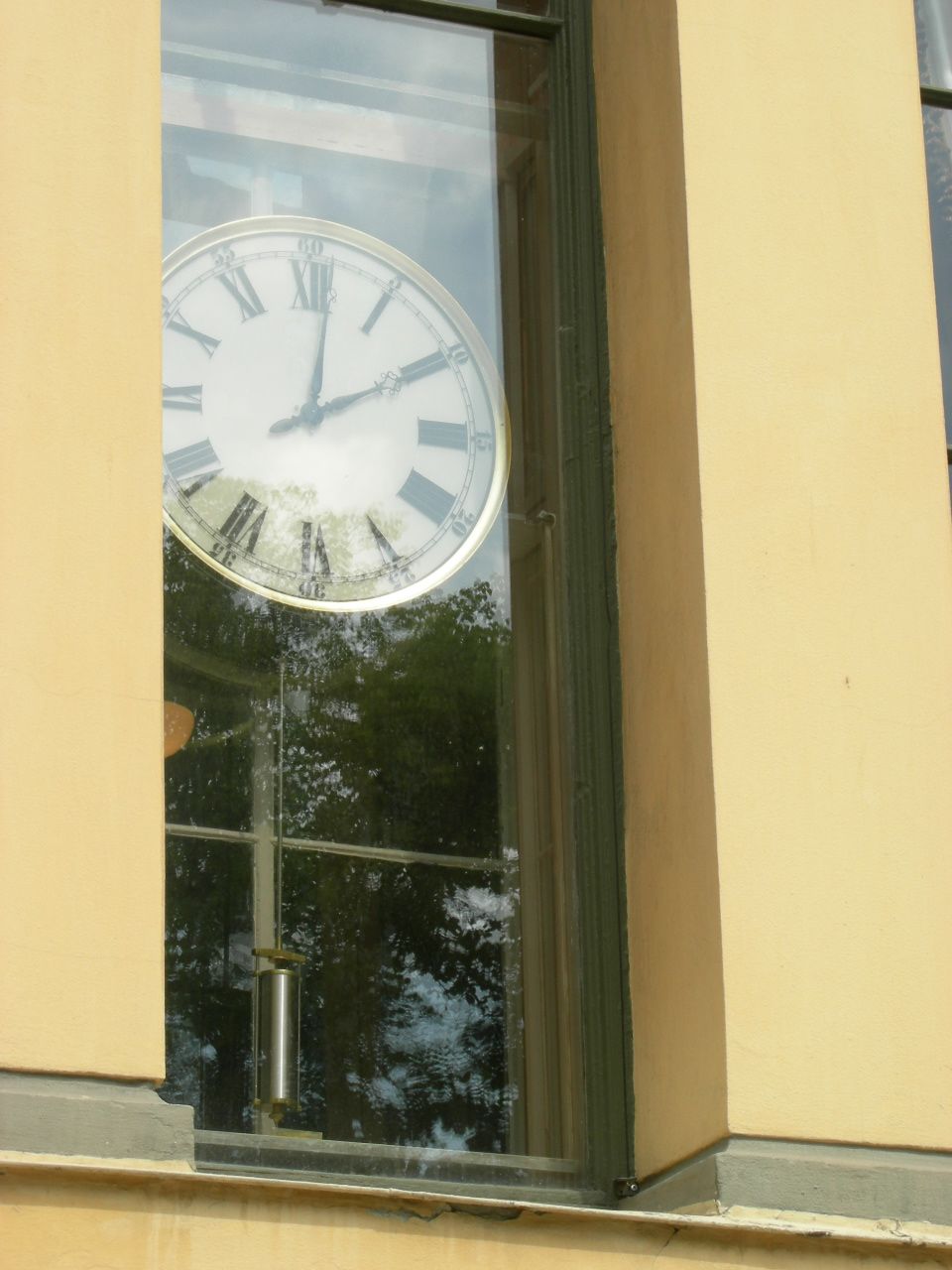The photograph captures a regular pane window set within a building with tan plaster walls. Dominating the upper half of the window is a silver clock with a pendulum extending downward. The clock's face is white and marked with elegant black Roman numerals, showing the time as 2 o'clock. The clock, whether wall-mounted or freestanding, remains indistinct. A noticeable glare on the window reflects images of trees and the sky, suggesting the photo was taken from slightly below eye level.